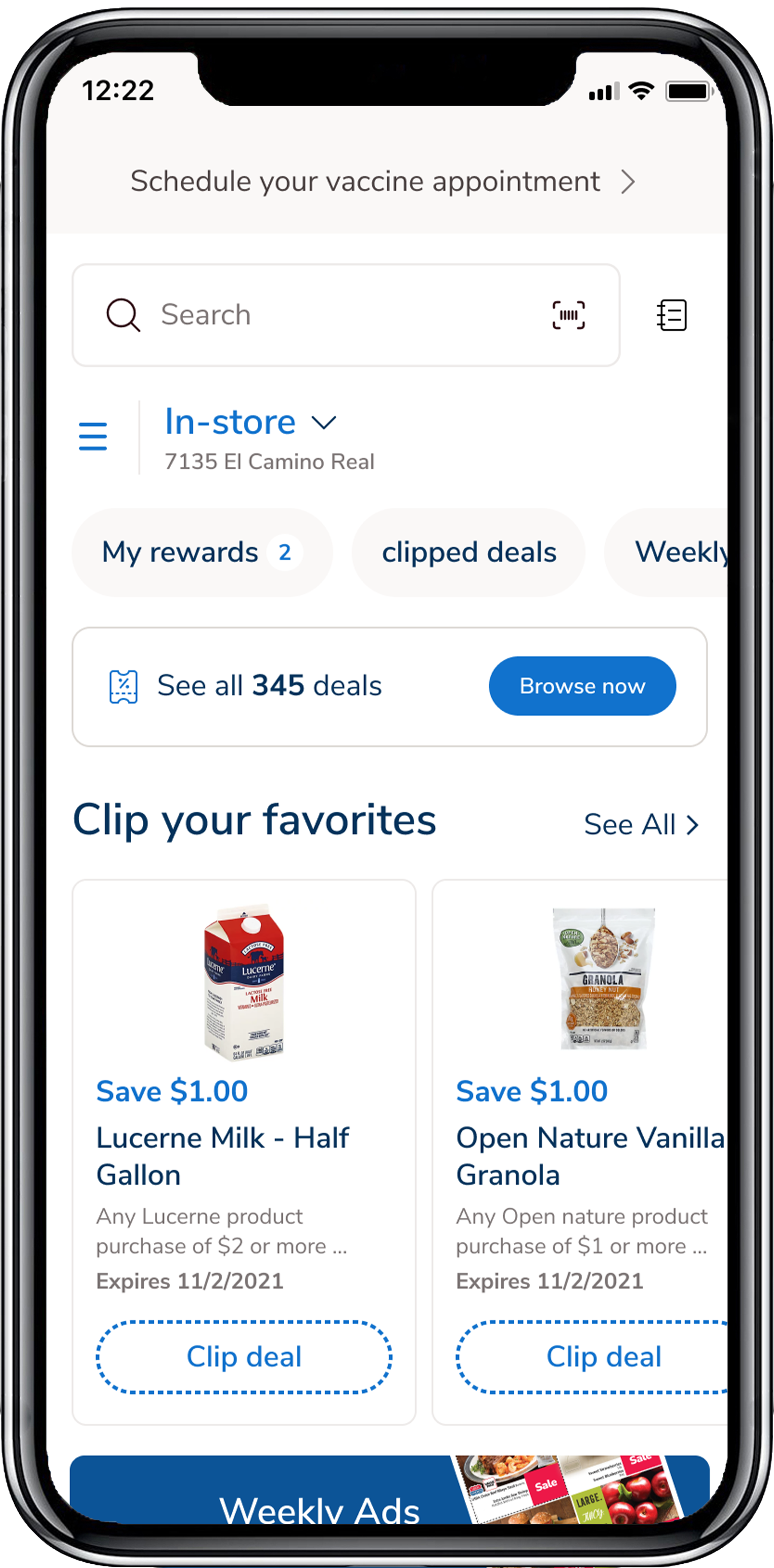The image showcases a smartphone with a website displayed on its screen. The phone has a sleek silver exterior with a black inner border. At the top center of the screen, there is a small notch for the front camera. The phone's status bar indicates the time as 12:22 PM, with icons for battery life, Wi-Fi connection, and internet signal on the right.

Below the status bar, a banner reads, "Schedule Your Vaccine Appointment," with an arrow pointing to the right. Beneath this, there's a search bar with a notebook icon adjacent to it. On the left side, there are three horizontal blue lines, likely representing a menu button, followed by a dropdown menu labeled "In-Store." Next to this is an address field.

Further down, the screen features three gray tabs with black text. The first tab, labeled "My Rewards," shows a blue "2" badge. The second tab is labeled "Clip Deals," and the third tab, labeled "Weekly," extends off the screen to the right. Below these tabs is a rectangular section containing a square with an 'X' inside, accompanied by a message indicating the presence of 345 deals. A prominent blue button within this section says "Browse Now" in white text. 

Another section titled "Clip Your Favorites" appears below, with an option to "See All" on the right. To the left, there is a picture of two items. The first item is a carton of Lucerne Milk, featuring red, blue, and white colors, along with the text "Save $1 Lucerne Milk - Half Gallon." Detailed information is listed beneath, along with a blue "Clip Deal" button. The second item is a package of vanilla granola, presented similarly with detailed savings information.

At the very bottom, just barely visible, is the top portion of a blue banner reading "Weekly Ads."